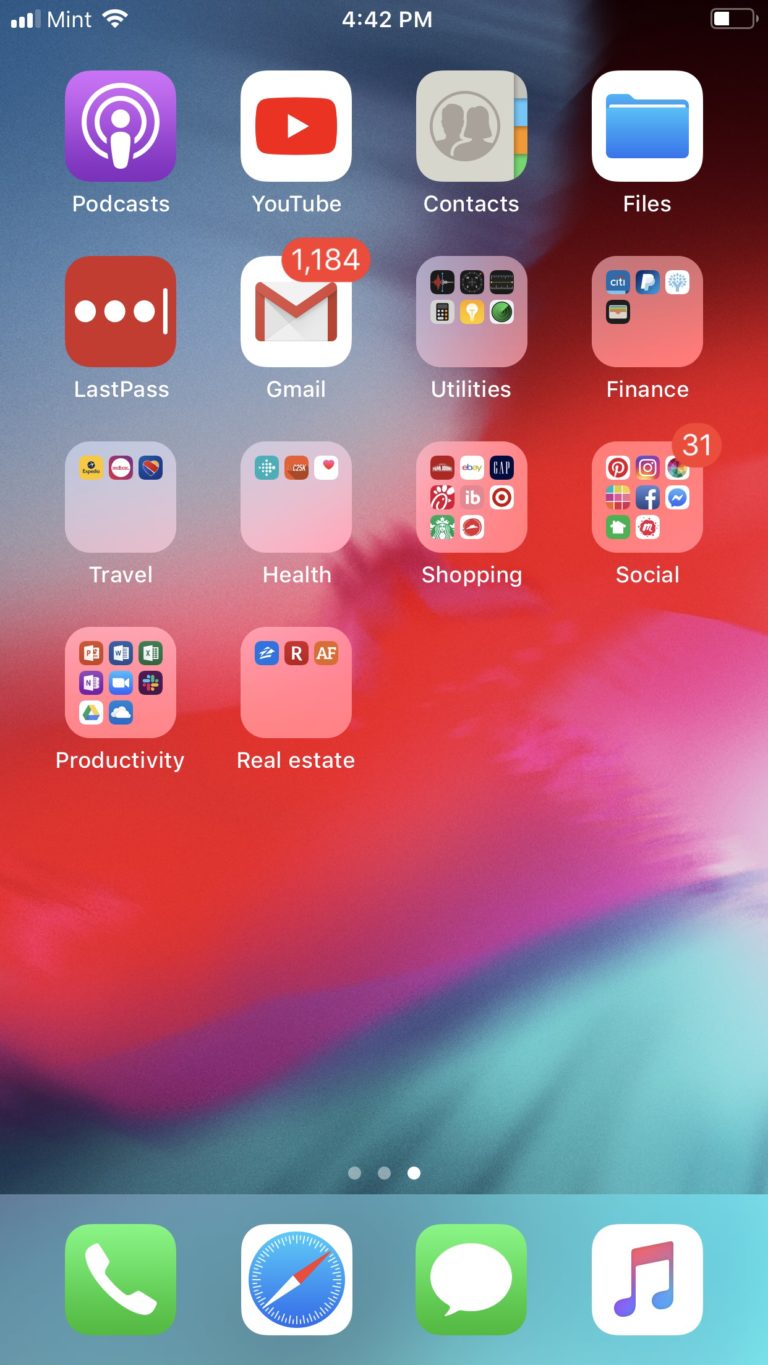The image showcases a busy smartphone home screen filled with a variety of app icons and folders, set against a background with slight paint splotches in pink, red, and blue.

The top left corner features a purple square labeled "Podcast" and a white square with a YouTube symbol. Adjacent to them is a gray square, a white square with a blue file folder labeled "Files," and a red square containing three white circles identified as "LastPass."

Below these, there is a Gmail icon with an envelope symbol. A red circle labeled "1184 utilities" hosts six different apps. The screen also contains folders named Finance (with four apps), Travel (with three apps), Health (with three apps), Shopping (with eight apps), and Social (with eight apps).

Additionally, there is a red circle indicating "31," containing a Productivity folder with eight apps and a Real Estate folder with three apps.

Towards the bottom of the screen, there are three circles. The third circle, being white, includes a green square with a white phone icon, a Safari symbol, a green square with a white chat icon, and a white square with a music note in red, blue, and purple colors.